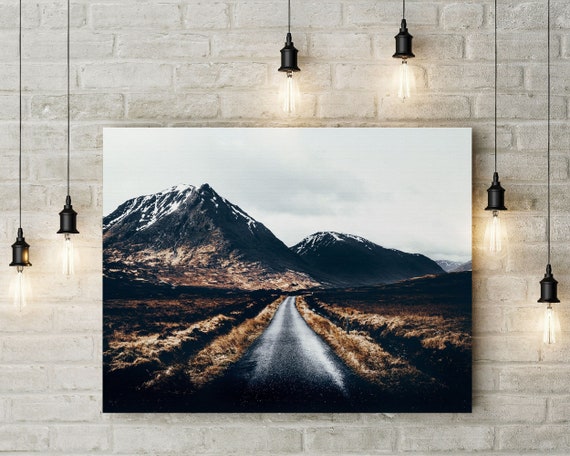A detailed photograph print hangs on a white brick wall, surrounded by six randomly placed pendant lights. The composition of the hanging lights—two on the left, two on the right, and two at the top—adds an eclectic symmetry to the scene. The photo itself, printed on canvas, depicts a straight, well-paved road stretching through dry, brown plains towards a distant mountainous horizon. The mountains, dark and rocky at the base, transition to snow-capped peaks under an overcast, gray sky. The low vegetation along the road's sides adds muted tones of brown, cream, and the occasional dark patch, enhancing the high contrast filter of the image.